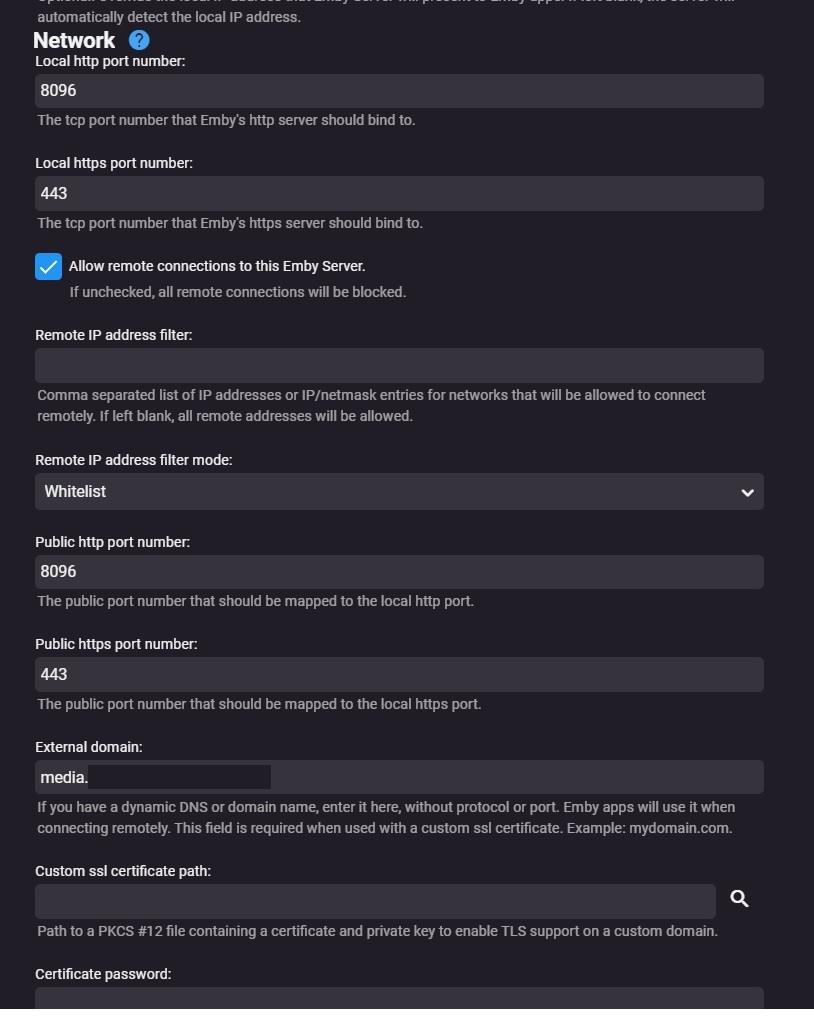**Screenshot Description: Settings Interface for MB Server Configuration**

The background of the screenshot is entirely black. At the top, the text is partially obscured, with only the second line visible. The visible text reads: "Automatically detect the local IP address," with "IP" in uppercase letters.

Following a small gap, there is a heading in bright white print: "Network" with a capital "N". Adjacent to this heading, there's a blue circle containing a black question mark.

Below, it reads "Local HTTP port number" which is specified as "8096." Beneath this, it states: "The port number that MB's HTTP server should bind to," with "MB" in uppercase letters.

Next, it specifies "Local HTTPS port number" as "443," followed by: "The TCP port number that MB's HTTPS server should bind to."

Further down, there is a blue square with a white check mark inside. It includes the text: "Allow remote connections to this MB server. If unchecked, all remote connections will be blocked."

The next section lists "Remote IP address filter" and "Remote IP address filter mode" followed by "Whitelist."

For public access, it specifies:
- "Public HTTP port number: 8096"
- "Public HTTPS port number: 443"

The description continues with "External domain media," followed by more text that is cut off. Lastly, it mentions "Custom SSL certificate path" followed by "Certificate password," with this part also cut off.

(Note: "MB" presumably refers to a specific media server, though the exact name is not fully visible. Details on certain settings and their implications are explained, suggesting it's part of an advanced configuration interface for a server application.)